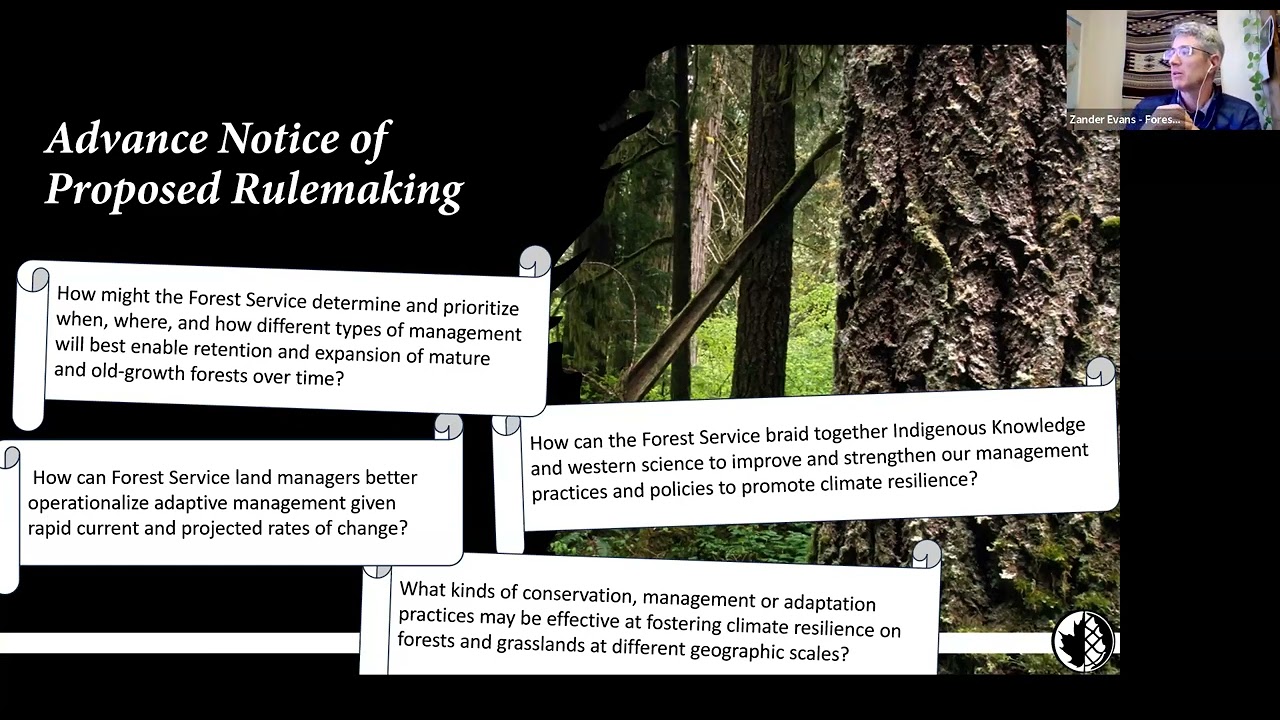This detailed colored image, resembling a slide from an online presentation, features a black background with a title in white text on the top left reading "Advanced Notice of Proposed Rulemaking." The slide is divided into two main vertical sections. The left section is primarily text-focused, displaying four important queries in text boxes formatted like scrolls:

1. How might the Forest Service determine and prioritize when, where, and how different types of management will best enable the retention and expansion of mature and old-growth forests over time?
2. How can Forest Service land managers better operationalize adaptive management given rapid current and projected rates of change?
3. How can the Forest Service braid together Indigenous knowledge and Western science to improve and strengthen our management practices and policies to promote climate resilience?
4. What kinds of conservation management or adaptation practices may be effective at fostering climate resilience on forests and grasslands at different geographic scales?

On the right side, a detailed image of tree trunks with lush green grass in the background provides a naturalistic visual contrast to the text. Below the scrolls, near the bottom edge of the slide, a small, round black-and-white logo appears, featuring an intricate design that seems to merge a Canadian maple leaf and a pine cone.

In the upper right-hand corner of the slide, within a smaller rectangular window—a picture-in-picture format—the presenter, identified as Xander Evans, is visible. He is a white male with gray hair, glasses, and earbuds, suggesting he is giving a live online presentation, probably through a Zoom meeting. The combination of visuals and content provides a comprehensive overview of proposed forestry management initiatives and invites active audience engagement through thought-provoking questions on environmental management practices.